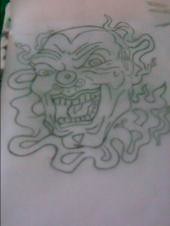This is a highly detailed black and white tattoo drawing featuring a horror-themed clown. The clown is visually striking with an ominous and unsettling appearance. Its face is adorned with exaggerated features, including a very round nose and an unnervingly wide grin that reveals large, menacing teeth reminiscent of the Joker's smile. The eyes are large and piercing, framed by raised eyebrows that enhance the sinister expression. A dark outline accentuates the typical areas where white makeup would be, creating a stark contrast. Emerging from the clown's head are serpentine shapes that resemble snakes, adding to the grotesque and eerie atmosphere of the image. The clown's facial structure is further defined by prominent cheeks and a pronounced chin. Around its neck, the clown wears a ruffled collar, completing the macabre aesthetic of this intricately designed tattoo drawing.